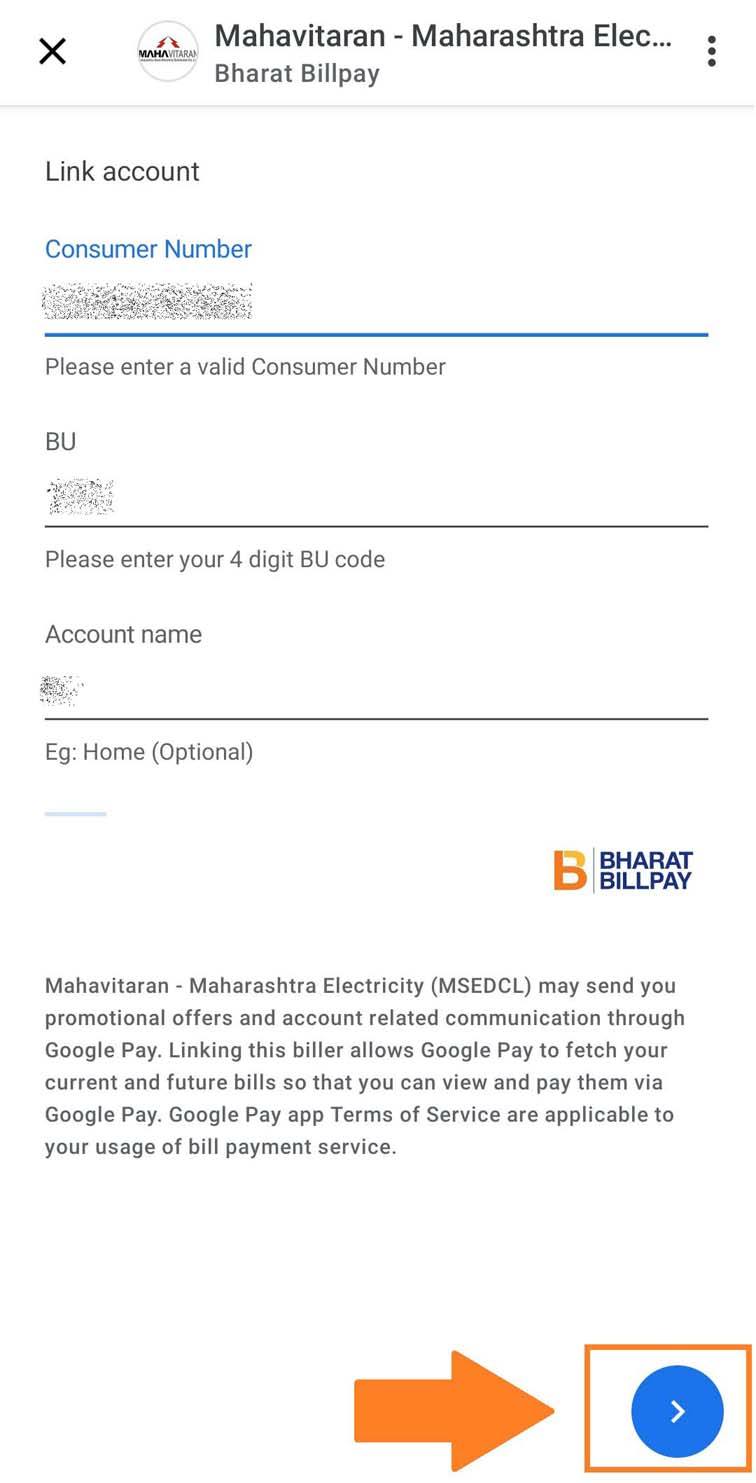This is a detailed screenshot from a cell phone interface, featuring a predominantly white background. In the upper left-hand corner, there's a gray "X" icon. Immediately to the right is a gray-outlined circle. Dominating the center of the image is a horizontal gradient line that transitions from dark gray to light gray. Above this line is a noticeable red half-circle. Adjacent to this red semi-circle, the text "MAHAVITARAN" in gray is prominently displayed, followed by "─ MAHARASHIRA" partially visible, and "ELEC..." truncated by ellipses.

Below these elements lies another light gray horizontal line. The next line of text reads "Link Account" in gray. Situated two lines below, the text "Consumer Number" appears in blue. Underneath this, a gray rectangle obscures additional information. A solid blue line extends horizontally beneath it, followed by the prompt "Please enter a valid consumer number" in gray font.

Approximately three lines further down, the screen displays the text "BU" in capital letters, next to a gray blocked-out square. Another black horizontal line appears below these elements. Further down, the instruction "Please enter your four-digit BU code" is displayed in gray text.

Moving down a couple of lines, the text "Account Name" appears in gray, followed by another black horizontal line. Beneath this, "EG: home (optional)" is written in gray text.

Towards the bottom right corner, there's an orange capital "B". To its right, the text "BHARATBILPAY" is written in black text. Below this, a paragraph of small light gray writing is present, albeit difficult to read due to its size and lightness. Finally, at the bottom right, there's a large filled-in arrow pointing to the right, and a square outlined in orange. Inside this square is a blue circle containing a white arrow oriented to the right, resembling a sideways "V".